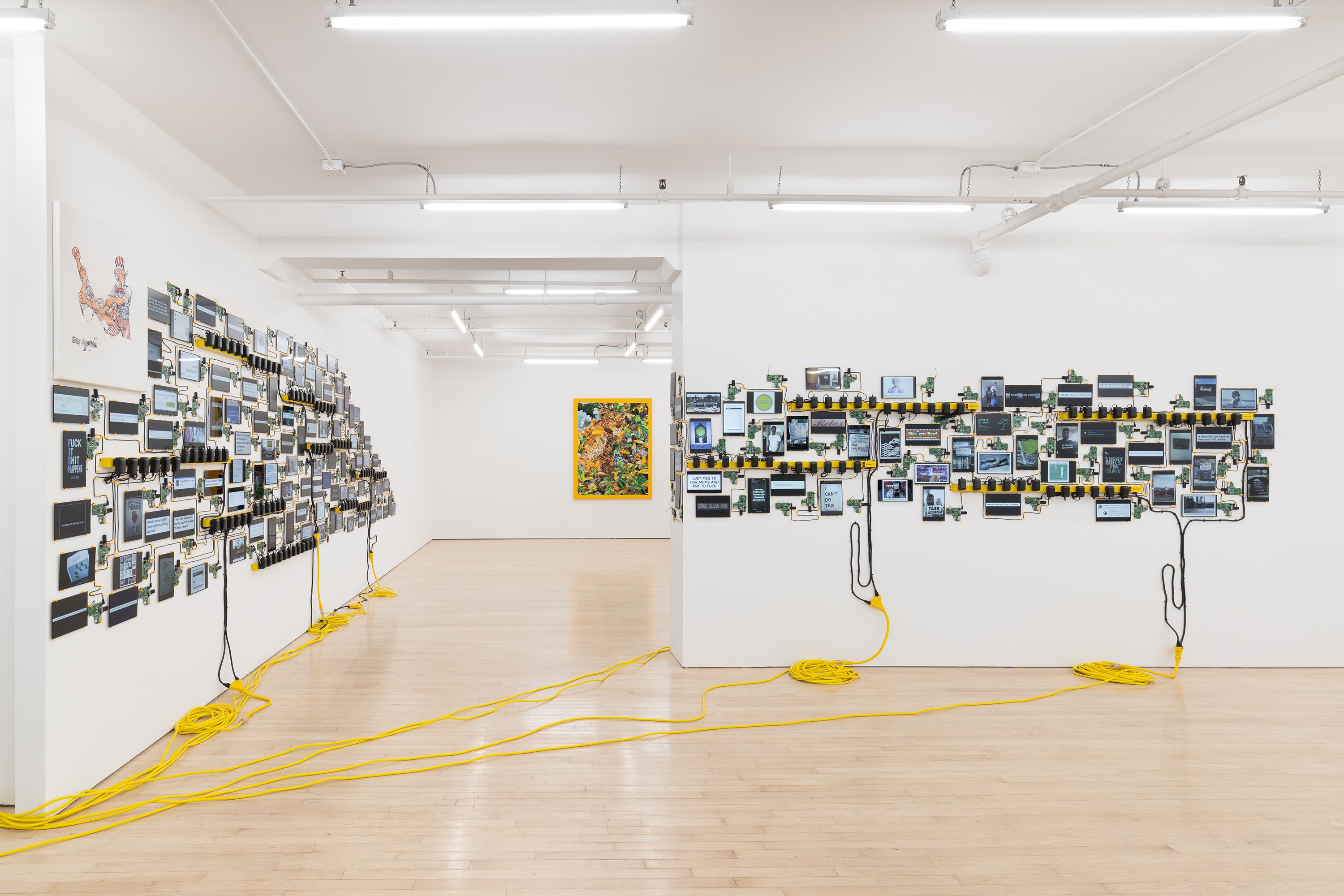The image depicts a brightly lit gallery installation within an art museum. The space features white walls and a light yellow wooden floor that appears reflective, capturing the gleam from overhead lights. Central to the installation are numerous tablets mounted on the walls. These tablets are uniform in size and display varied content on their screens. They are powered via interconnected yellow cables, converging into power strips positioned at the base of the walls. On the left wall, one hundred small screens, each slightly larger than a cell phone, are arranged in a grid-like pattern. A similar setup is observed on the right wall where the tablets are also connected by yellow wires. In the background, an abstract painting in a yellow frame hangs on the far wall, adding an additional layer of depth to the overall scene. Subtle details such as the placement of cords and the reflective quality of the floor enhance the immersive experience of the installation. There is no text present in the image, keeping the visual focus on the art and its structural elements.